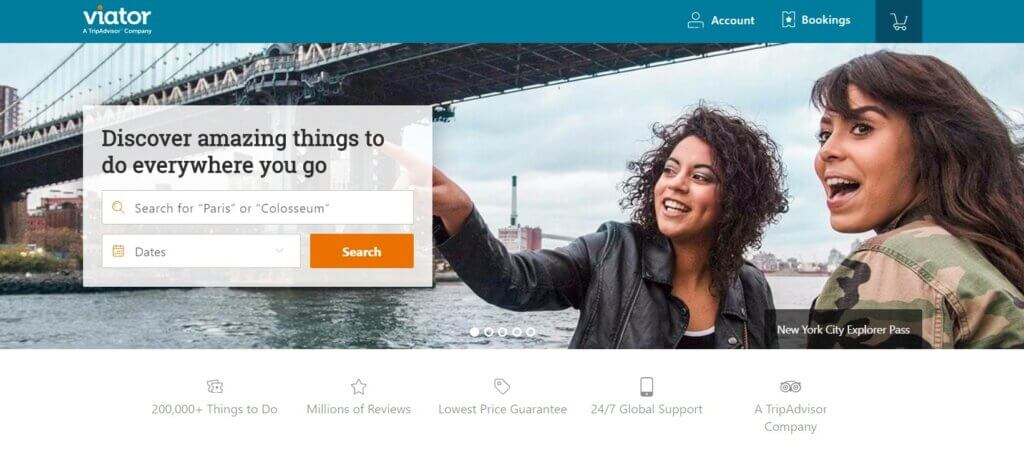The screenshot showcases a website named "BIATOR," with the site's name displayed prominently in white text against a blue background. Below the main heading, smaller white text, too small to discern, is visible. To the right of the site name, navigation options for "Account," "Bookings," and "Cart" are available for user interaction.

Beneath this navigation bar, there is a vivid image featuring two women situated in what appears to be New York City. They stand under a bridge, adjacent to a body of water. Both women have dark hair; one is dressed in a camouflage jacket while the other wears a leather jacket and is seen pointing to the left.

Overlaying this image is a prominent search box with the message "Discover amazing things to do everywhere you go." The search box allows users to input search terms and dates for planning activities.

Further down the page, textual highlights include:
- "200,000 things to do"
- "Millions of reviews"
- "Lowest price guarantee"
- "24/7 global support"
- A note indicating the site is a part of the "Tripadvisor" company family.